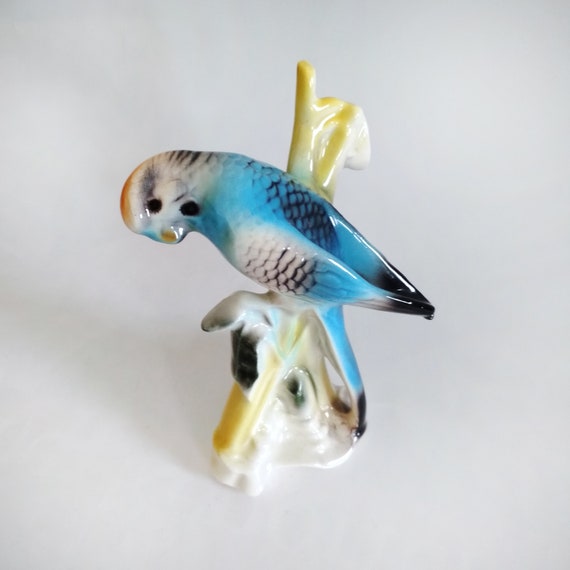This close-up color photograph captures a delicate ceramic figurine of a bird perched on a yellow and white tree branch, set against a stark white background. The bird, with its predominantly light blue body, gleams under the light, showcasing the shiny glaze that covers its surface. Its head is turned downwards, revealing a small orange beak and a black eye. The bird's face is primarily white with patches of black, and there's a hint of orange on the top of its head. The wing on the left side is white tipped with blue, while the tail feathers are black. The figurine closely resembles a finch or sparrow, merging elements of both porcelain and possibly blown glass, adding to its intricate and delicate appearance.